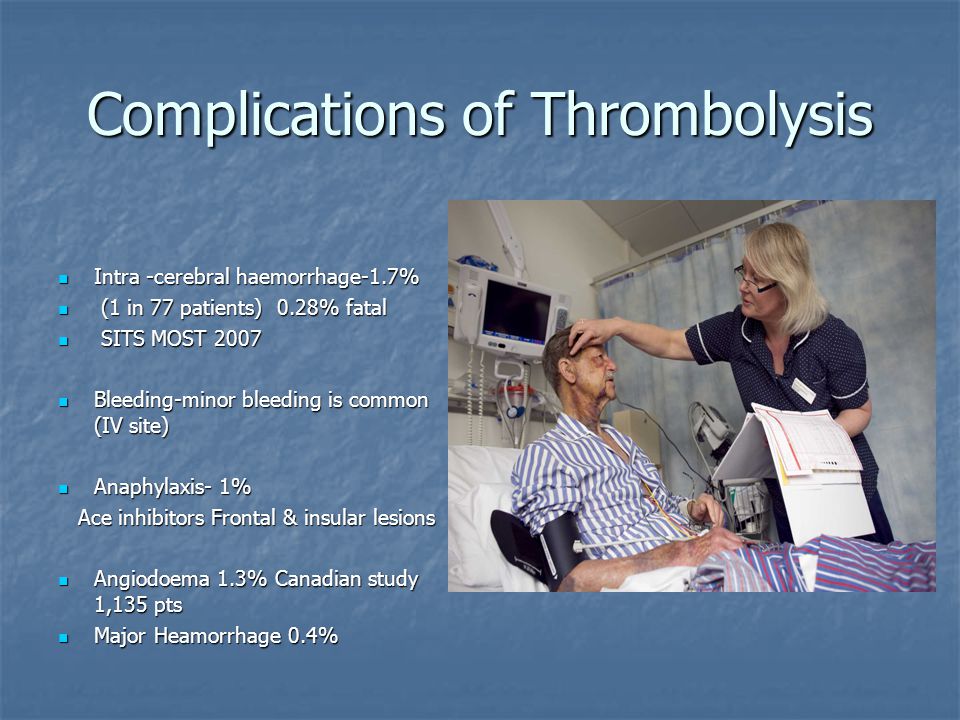The horizontal rectangular image appears to be a slide from a medical presentation, featuring a dark blue background. The heading at the top in large white letters reads "Complications of Thrombolysis." On the right side of the slide, there is a photograph of a patient in a hospital bed, wearing blue and white pajamas, with a red and blue blanket. A nurse, dressed in a dark blue dress, is attending to the patient, who is connected to a blood pressure cuff. She appears to be examining the patient's head or eyes, with bedclothes draped over her arm. There is also a medical monitor visible in the background.

On the left side of the slide, a series of detailed bullet points outline specific complications of thrombolysis along with their occurrence rates:
- Intracerebral hemorrhage: 1.7%, 1 in 77 patients, 0.28% fatal
- SITS-MOST 2007 study
- Bleeding: Minor bleeding is common at the IV site
- Anaphylaxis: 1%
- ACE inhibitors relevance
- Frontal and insular lesions
- Angioedema: 1.3%, Canadian study with 1,135 patients
- Major hemorrhage: 0.04%

Overall, the slide provides a detailed overview of potential complications associated with thrombolysis, supplemented by statistical data and visual context from the depicted hospital setting.